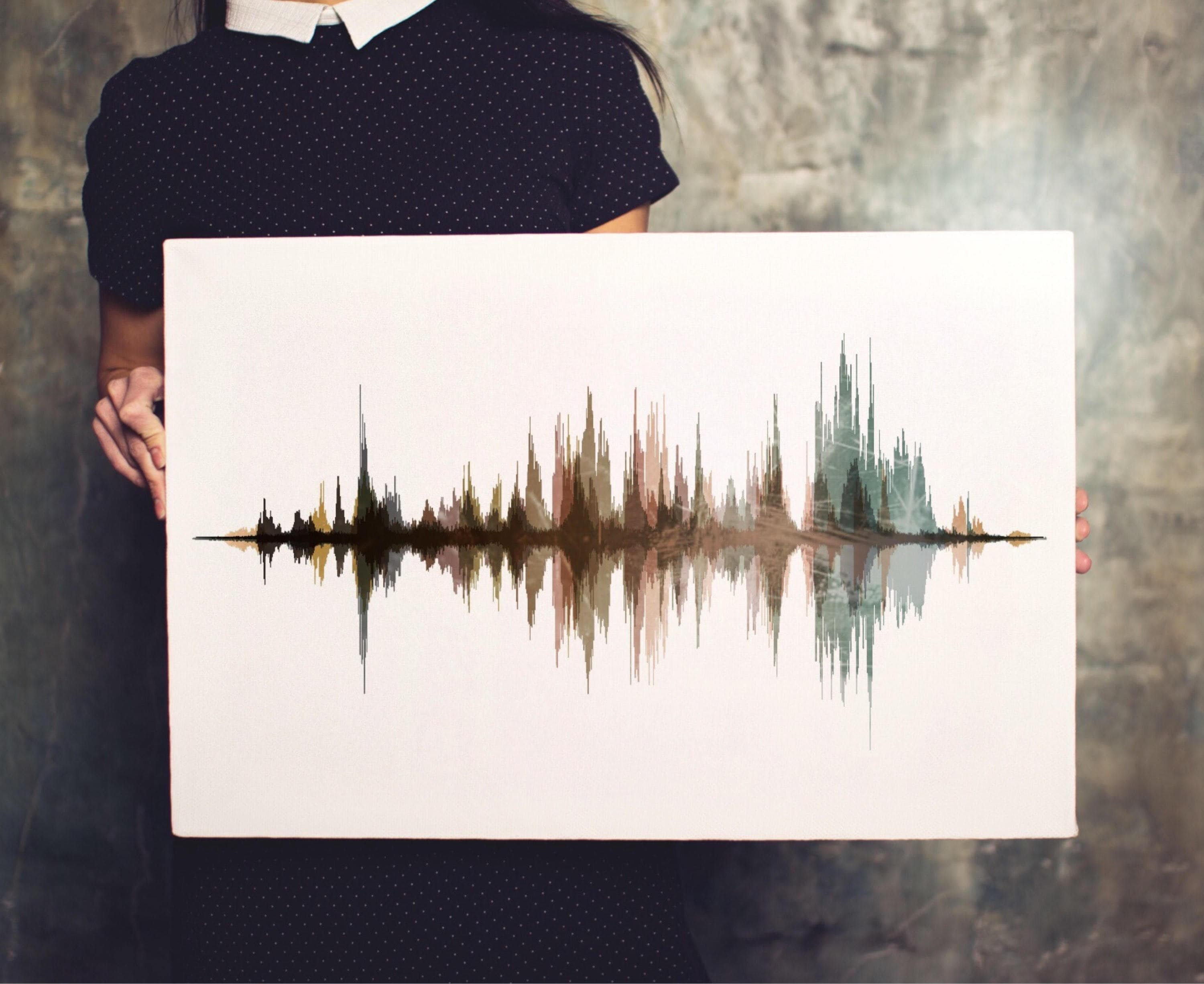This photo features a woman standing against a gray, splotched wall, holding a rectangular painting on a large white canvas. The woman, whose head is cropped out of the frame, has long dark hair and is dressed in a navy blue shirt with white dots and a white collar. The artwork she holds resembles a sound wave or a heartbeat graph, with a central horizontal line and numerous vertical lines extending above and below it. The lines vary in color and length, transitioning from black to dark brown, then light brown, reddish-brown, and finally dark green with hints of blue, creating an abstract, dynamic visual effect that evokes the feel of sound waves or abstract reflections. The setting is simple and modern, with the gray wall providing a neutral backdrop that accentuates the bold colors and intricate details of the painting.